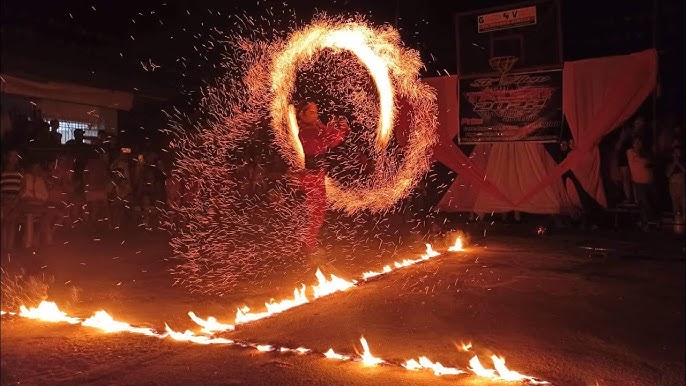This nighttime photo captures an outdoor festival featuring a fiery performance. At the center is a performer, likely male, clad in a red outfit, manipulating a fire prop that sends sparks flying in a circular pattern. Bright, flaming lines create a T-shaped formation on the ground, with one line running straight from left to right and another perpendicular line extending towards the background. The air is filled with glowing particles from the fire. In the backdrop, a sign possibly reads "2022." Crowds of spectators, some seated in white plastic chairs and others standing, are gathered around in the darkness, intently watching the dazzling pyrotechnic display.